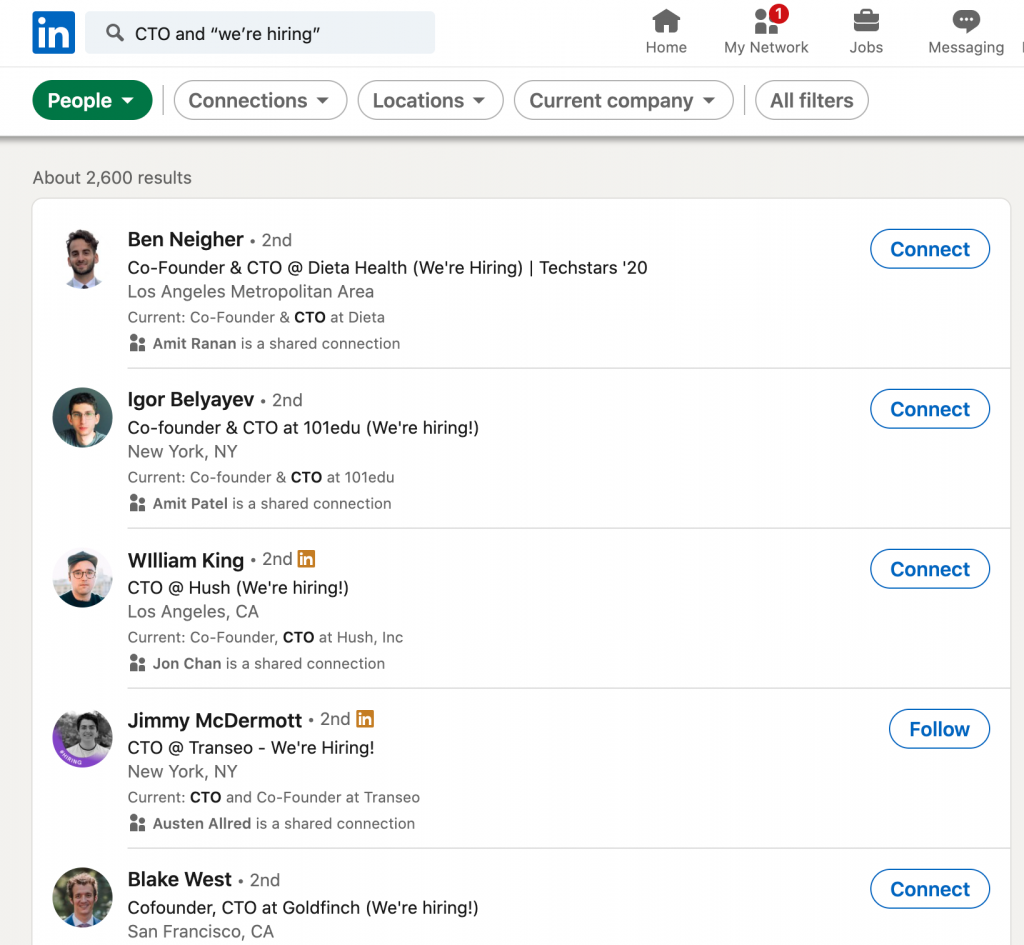A detailed and cleaned-up caption for the given image could be:

"Screenshot of a job search interface on a gray background featuring a search bar at the top. The search bar contains the text 'CTO (we're hiring)' in white text on a blue square, with a magnifying glass icon to the left. Below the search bar, there are several navigation tabs including 'Home,' 'My Network' with a red notification badge showing the number '1,' 'Jobs,' 'Messaging,' and 'Notifications,' displayed in a green oval with additional options like 'Connections,' 'Locations,' 'Current Company,' and 'All Filters.' The search results show approximately 2,600 listings.

The results are divided into five sections:

1. *First Listing:* Ben Neigher (Second-degree connection), Co-founder and CTO at Data Health (we're hiring), associated with Techstars, with a blue 'Connect' button.
2. *Second Listing:* Igor Belov (Second-degree connection), Co-founder and CTO at 101 Edu (we're hiring), also featuring a blue 'Connect' button.
3. *Third Listing:* William King (Second-degree connection), CTO at Hush (we're hiring), highlighted with an orange square.
4. *Fourth Listing:* Jimmy McDermott (Second-degree connection), showing an orange square similar to the previous listing.

Each entry displays a 'Connect' button in a blue oval to facilitate networking, emphasizing active recruitment for CTO positions by the companies listed."